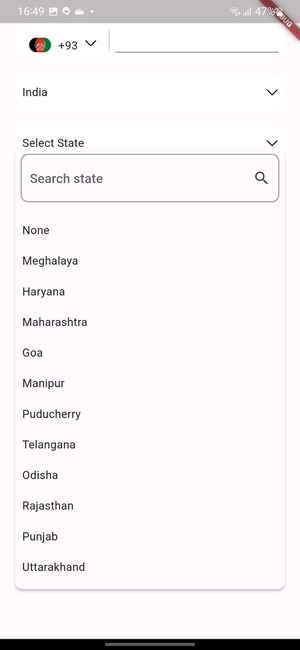The image showcases a screenshot of a website with various interface elements. 

At the top, there's a narrow, light gray banner featuring white text on the left that reads "16:49." Adjacent to this text, there's a small square icon depicting mountains with a dot above them, followed by additional graphic elements including a circle and a slightly blurred icon, culminating in a dot. 

On the right side of this gray banner, there are icons indicating cell signal strength, WiFi signal, and battery life at 47%. 

Directly beneath this, there is a reddish-burgundy banner that overlays part of the gray banner, which contains the word "DEBUG" in white, vertically oriented text.

Following this, the main content is displayed against a white background. In the center, there's an oval shape divided into three sections: black on the left, red in the middle, and green on the right. Below this oval, it reads "+93" with a downward arrow.

The next section features the word "India" with a downward arrow symbol next to it. Below "India," the text "Select State" appears with another downward arrow aligned to the right. 

Following this, there's a search bar with the placeholder text "Search state" accompanied by a magnifying glass icon. 

Below the search bar is a list of states and regions, starting with "None" and continuing with:

- Meghalaya (spelled as M-E-G-H-A-L-A-Y-A)
- Haryana (H-A-R-Y-A-N-A)
- Maharashtra (M-A-H-A-R-A-S-H-T-R-A)
- Goa
- Manipur
- Puducherry
- Telangana
- Odisha
- Rajasthan
- Punjab
- Uttarakhand